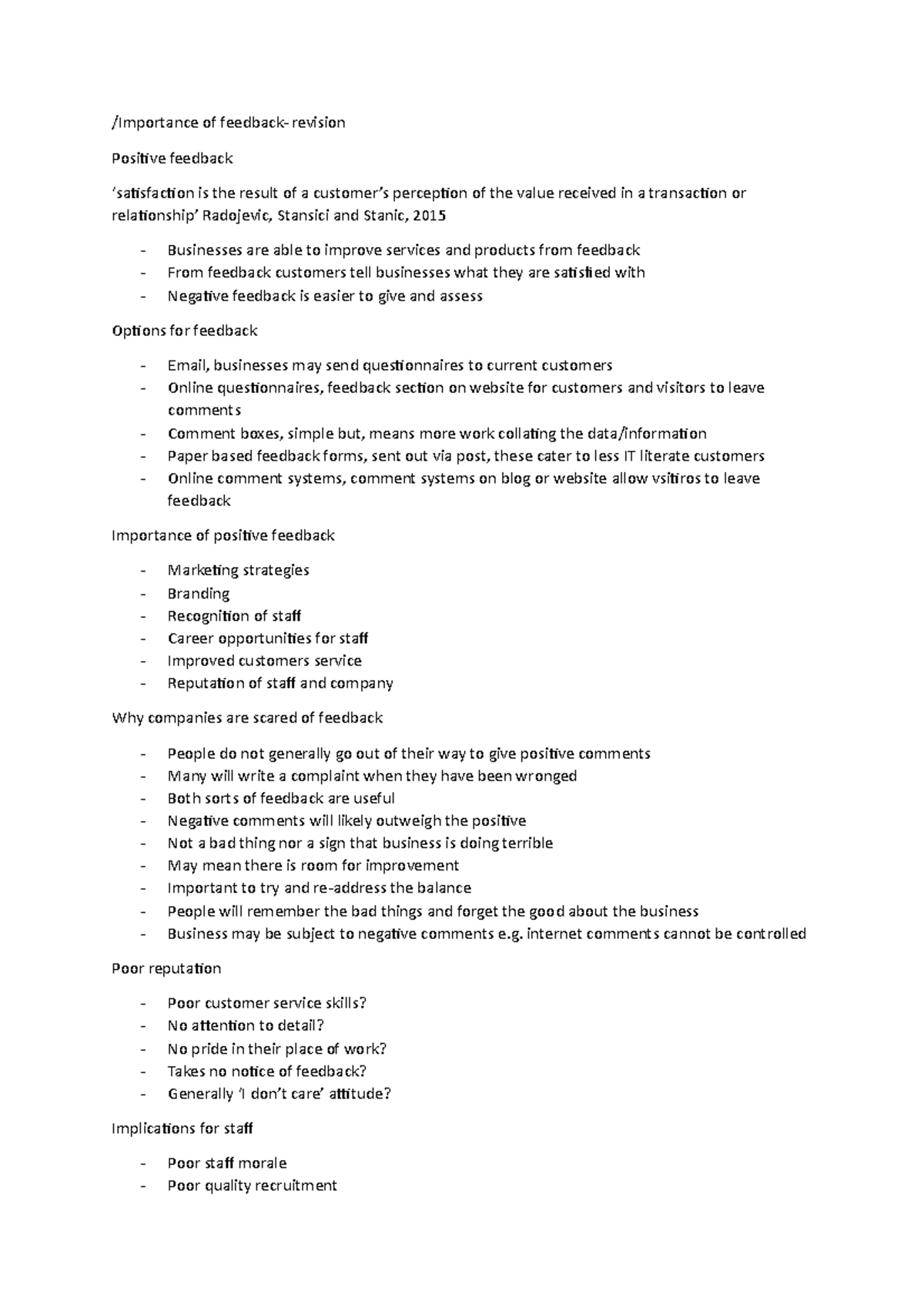The image illustrates various types of customer feedback mechanisms and their impact on businesses. It highlights the importance of collecting and analyzing feedback, both positive and negative, to enhance customer satisfaction and improve service delivery. The image depicts methods such as email questionnaires, online feedback forms, and paper-based feedback forms, emphasizing how each method allows customers to share their experiences and suggestions.

Key points include:

1. **Positive Feedback:** Customers providing positive feedback often express satisfaction with the value added to the product or service. This feedback helps businesses understand what they are doing right and encourages them to continue those practices.

2. **Negative Feedback:** Negative feedback, though easier for customers to articulate, provides critical insights into areas needing improvement. This type of feedback is essential for businesses to address issues promptly and prevent further dissatisfaction.

3. **Feedback Methods:** The image showcases various feedback collection methods:
   - **Email Questionnaires:** Targeted at current customers to gather comprehensive insights.
   - **Online Comment Sections:** Allow customers to leave feedback directly on websites or blogs.
   - **Feedback Boxes:** Simple yet effective for in-person feedback collection.

4. **Importance of Feedback:** Effective feedback collection and analysis can lead to improved marketing strategies, better branding, and recognition of career potentials within the company. Companies that actively seek and respond to feedback are more likely to maintain high customer satisfaction and loyalty.

5. **Implications of Neglecting Feedback:** Ignoring feedback can lead to negative consequences such as poor reputation, lack of attention to detail, and diminished pride in the business' work. This neglect can result in decreased staff morale, poor recruitment quality, and overall decline in service quality.

Overall, the image conveys the critical role of customer feedback in fostering a positive transaction relationship and enhancing the overall customer experience.